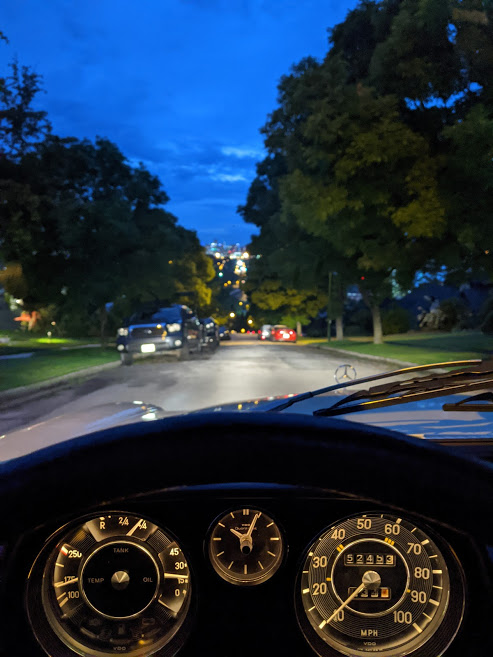This image captures a scene from inside a moving Mercedes-Benz car, with the focus through the steering wheel and across the partially visible hood, out onto a dimly lit street. It’s nearly dark, evident from the illuminated headlights and the lit gauges on the dashboard, which include a speedometer showing 10 miles per hour, an odometer reading 52453, a fuel gauge indicating more than three-quarters full, and an analog clock displaying 10:05. The street, lined with parked cars on both sides, is bordered by mown green grass and large trees under a cloudy, darkening sky. The city's lights can be faintly seen in the distance, enhancing the twilight ambiance of the scene.